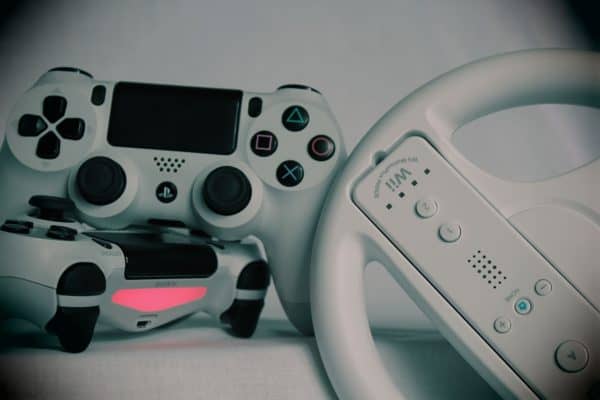This image portrays a collection of video game controllers set against a vignette-style backdrop, with the corners fading into darkness. The central focus includes two PlayStation controllers and a Wii accessory. On the right side, a white Wii remote is embedded in a matching white steering wheel, positioned upside down at an angle. The Wii remote features white buttons with black symbols, and a distinctive blue light on the middle button of a horizontal row. To the left, a white PlayStation controller rests upright atop another PlayStation controller, which lies flat. The upright controller exhibits the iconic PlayStation square, triangle, circle, and X buttons, with black analog sticks and directional buttons. The controller beneath it is largely obscured but presents a glowing red or pink stripe near the top. The predominantly white aesthetic of the controllers contrasts with the black and fading dark corners of the image, emphasizing the hardware's details amidst the low-light setting.